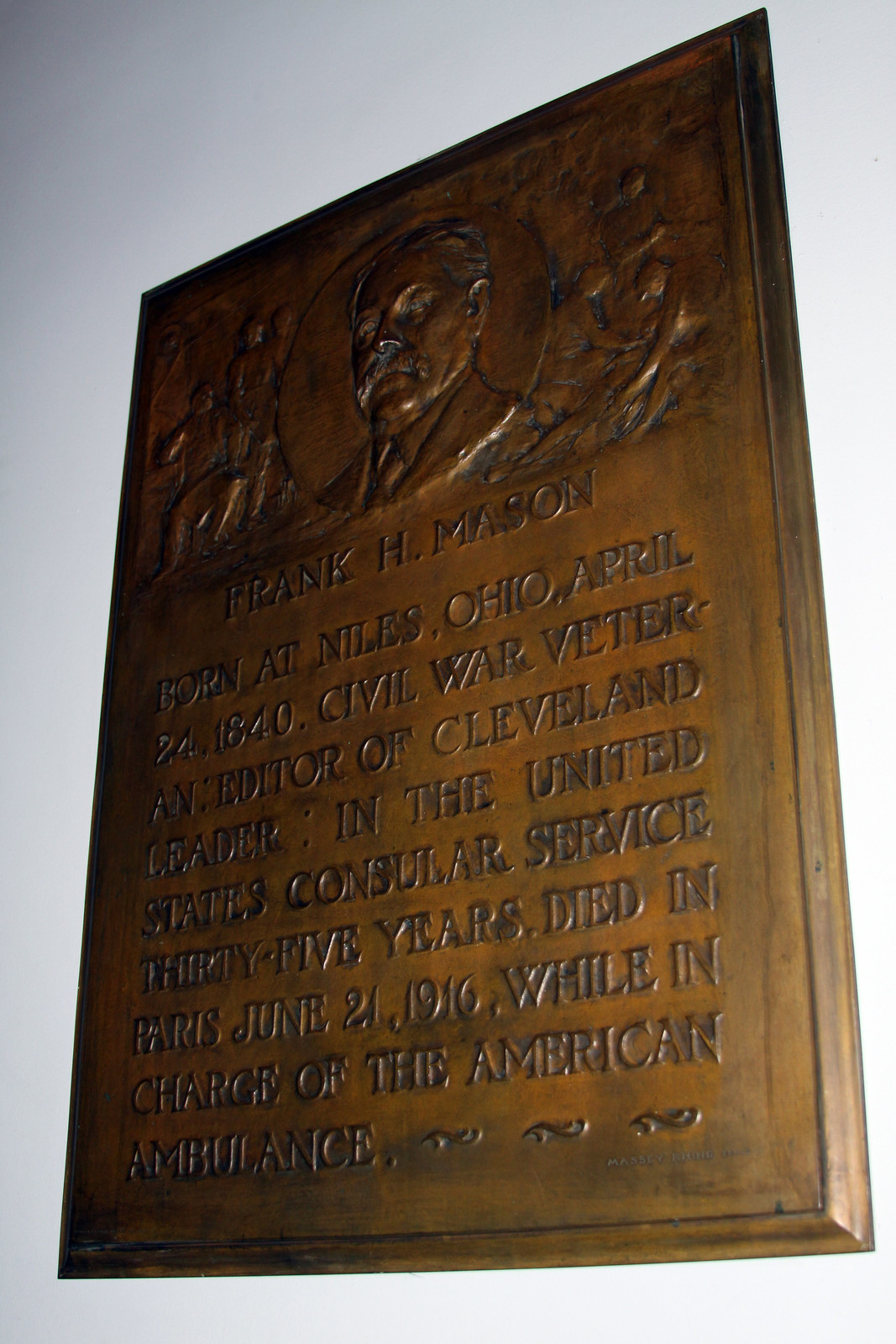This vertically oriented photograph captures a bronze plaque positioned against a white wall, seemingly taken indoors. The plaque exhibits a rectangular shape with beveled edges and features a central circular area containing a detailed bust engraving of a man named Frank H. Mason. The engraved bust shows Mason with short hair, a mustache, and wearing a suit. Surrounding the circular area are intricate carved decorations. Below the bust, an inscription details Mason's life: "Frank H. Mason, born at Niles, Ohio, April 24, 1840, Civil War veteran, editor of Cleveland Leader, in the United States Consular Service for 35 years, died in Paris June 21, 1916, while in charge of the American Ambulance." The background wall appears variably gray and white, likely due to the camera's lighting.